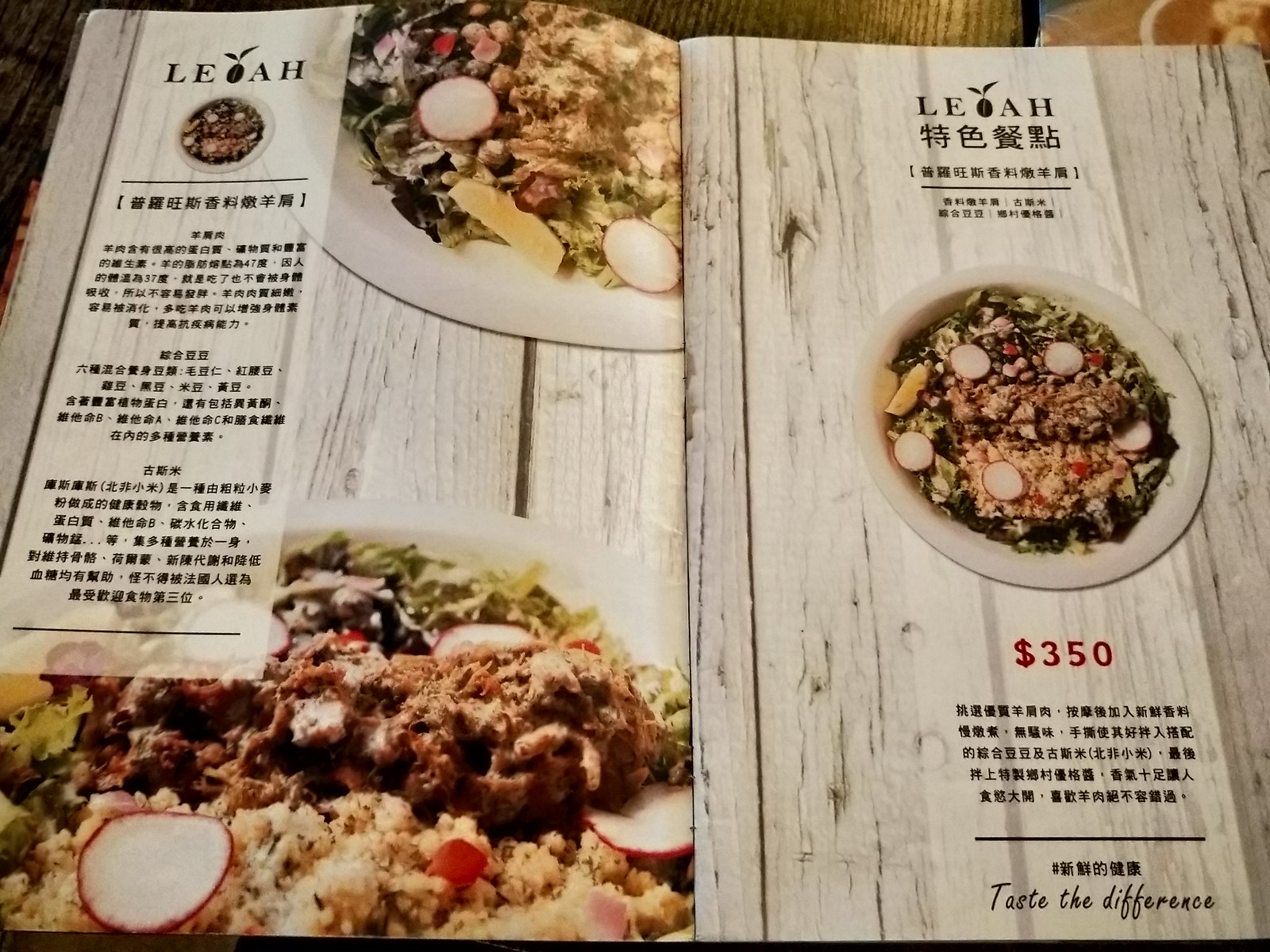The image depicts an open, professionally printed and laminated menu that appears to be from an upscale Asian restaurant. The menu's cover prominently displays the name "Lee Ah" alongside a shape resembling a pineapple. The menu consists of two visible pages, laid open in a book-style format.

On the left page, there are detailed pictures of a specialty dish. The images feature a beautifully presented meal with slices of radish, mixed meat, rice, sauce, and assorted vegetables. One image provides a closer view to highlight the intricate details of the dish, while the other shows the dish in its entirety, demonstrating its presentation on the plate.

The left page also features extensive text, presumably describing the dish and its ingredients, written in an Asian language. This detailed description signals the menu's target audience is one that appreciates a thorough understanding of their dining experience, which is characteristic of an upscale establishment.

On the right page, the same dish is showcased again in a full-plate view, centered on the page. Below the image, the price is listed as $350, which suggests this could either be an extraordinarily high-priced dish or might be indicative of a local currency value expressed with a dollar sign. More descriptive text is present both above and below the image, further emphasizing the significance of this specialty dish to the restaurant.

The bottom of the right page bears a tagline in an elegant English script font: "Taste the difference," the only fully readable English phrase besides the restaurant's name "Lee Ah."

The entire menu is set against a background that mimics distressed wood planks, likely enhancing the aesthetic appeal and subtly indicating the rustic yet refined atmosphere of the restaurant. This faux wood plank design might also be the surface on which the dishes were photographed.